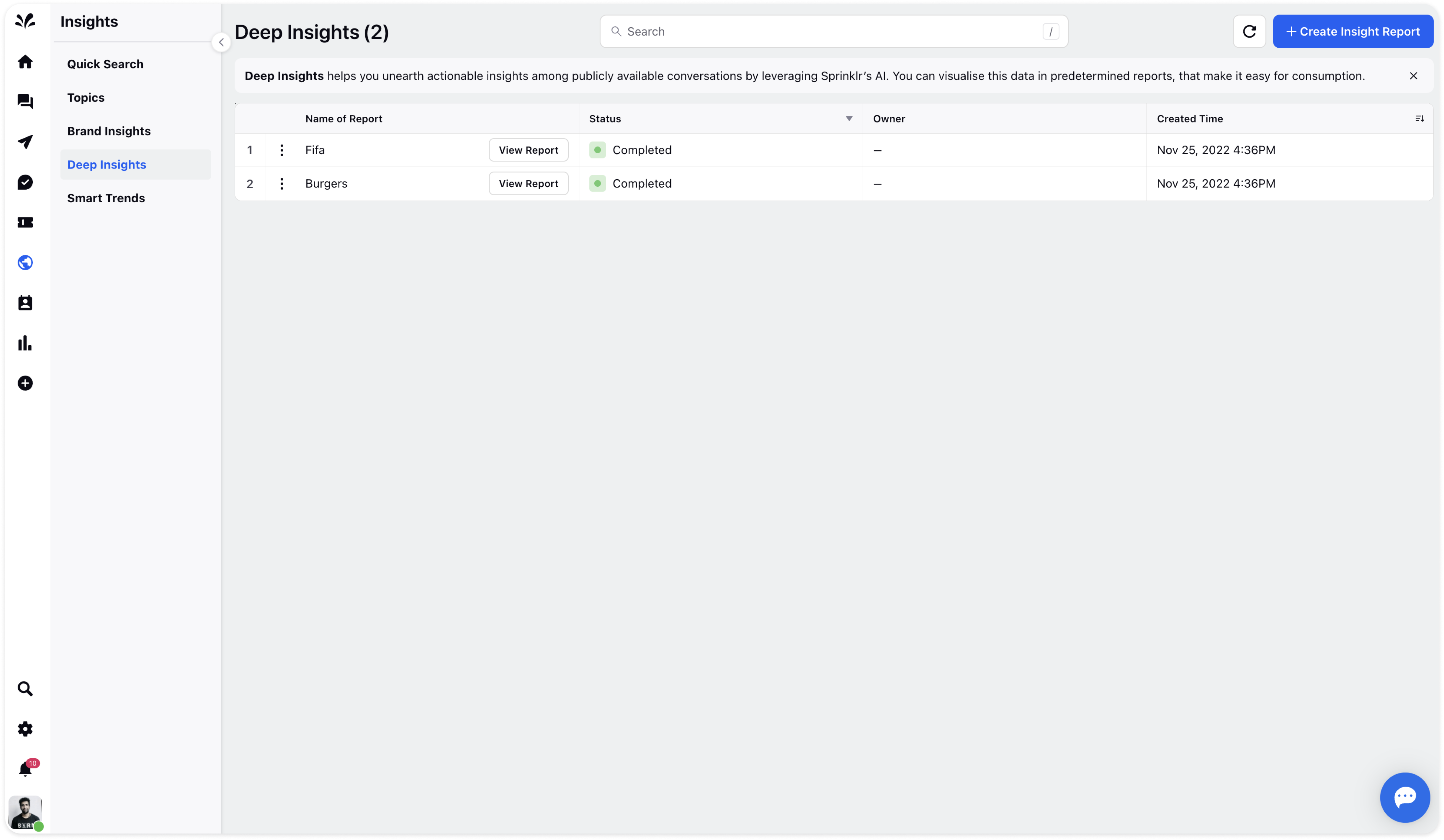On the "Insights" page, there's a detailed interface composed of several sections. On the bottom left, a small icon depicts a user profile, which appears to be a younger, Middle Eastern man. To the right of the icons, a pane titled "Quick Search Topics" lists various options such as "Brand Insights," "Deep Insights," and "Smart Trends," with "Deep Insights" currently selected.

The main section of the screen features a predominantly gray background with a list displaying two items: "FIFA" and "Burgers." Above the list is a description explaining that "Deep Insights" leverages Sprinklr's AI to unearth actionable insights from publicly available conversations. This data can be visualized in predefined reports for easier consumption.

A prominent blue button labeled "Create Insight Report" is situated at the top right, suggesting the ability to generate new reports. Below this button, it's indicated that reports on "FIFA" and "Burgers" have already been created, completed on November 25th, 2022, likely involving data compiled from various databases.